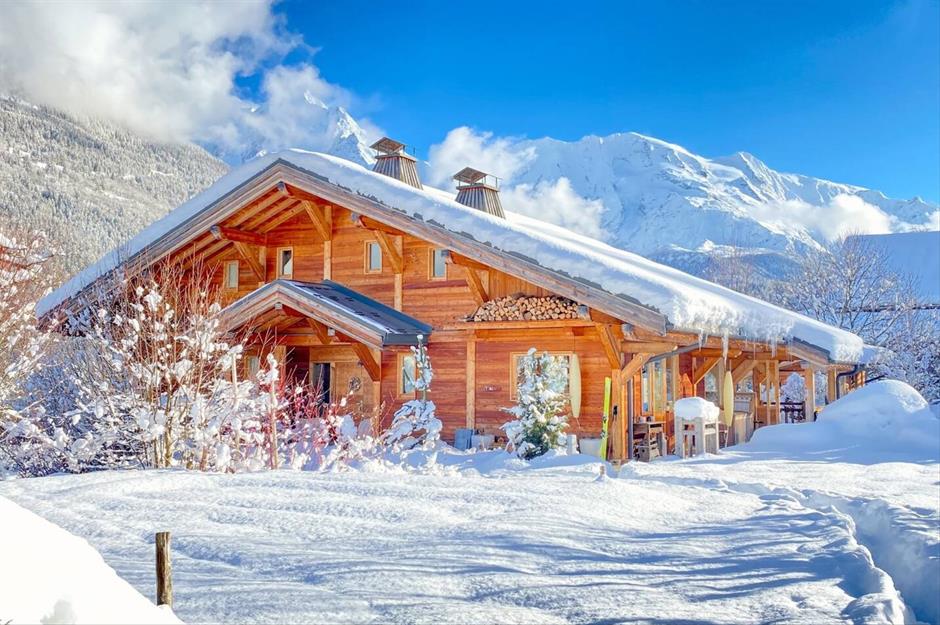In this photograph, a picturesque winter landscape showcases a light-colored wood cabin standing majestically in front of a stunning snow-covered mountain range. The cabin, captured from a frontal view, features a peak roof blanketed with a thick layer of snow and icicles beginning to form along the edges. On the outside, above one window, neatly stacked logs are visible on a shelf. The cabin's structure includes several windows—approximately four on the upper level, one on the lower level, and additional windows along the sides.

The surrounding area is a wintry paradise; barren trees, their branches laden with clumps of snow, encircle the cabin, adding to the serene ambiance. The ground is enveloped in a carpet of pristine, glittering white snow, which extends into the background where the towering, snow-coated mountains loom under a brilliant blue sky. To the right of the cabin, there is an open area with tables beneath the roof's overhang. Poles stand in front of the cabin beside the closed entrance door. The clear, sunny day casts a delightful contrast, with the sunlight shimmering off the snow, enhancing the beauty of this tranquil and secluded winter retreat.